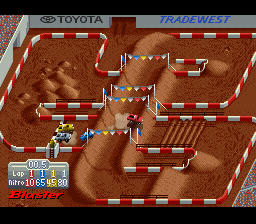This is a photograph of a video game focused on monster truck racing. In the bottom left corner, red letters display the word "Blaster," with a timer showing 5 seconds. The game appears to be in its first lap, indicated by "Lap 1/1/1." The nitro levels for the trucks are listed from left to right as 10, 65, 45, and 80.

The track resembles a dirt arena designed for monster trucks, with Toyota written on the left side of the inside wall and Tradewest on the right side. The image depicts two monster trucks parked in designated spots, ready for action. Surrounding parts of the road are red and white streamers, which likely serve as guardrails to keep the trucks on course. The scoreboard shows details such as the current timer at 5 seconds and the lap as "Lap 1/2/3." The nitro levels for the trucks are reiterated as 10, 65, 45, and 80.